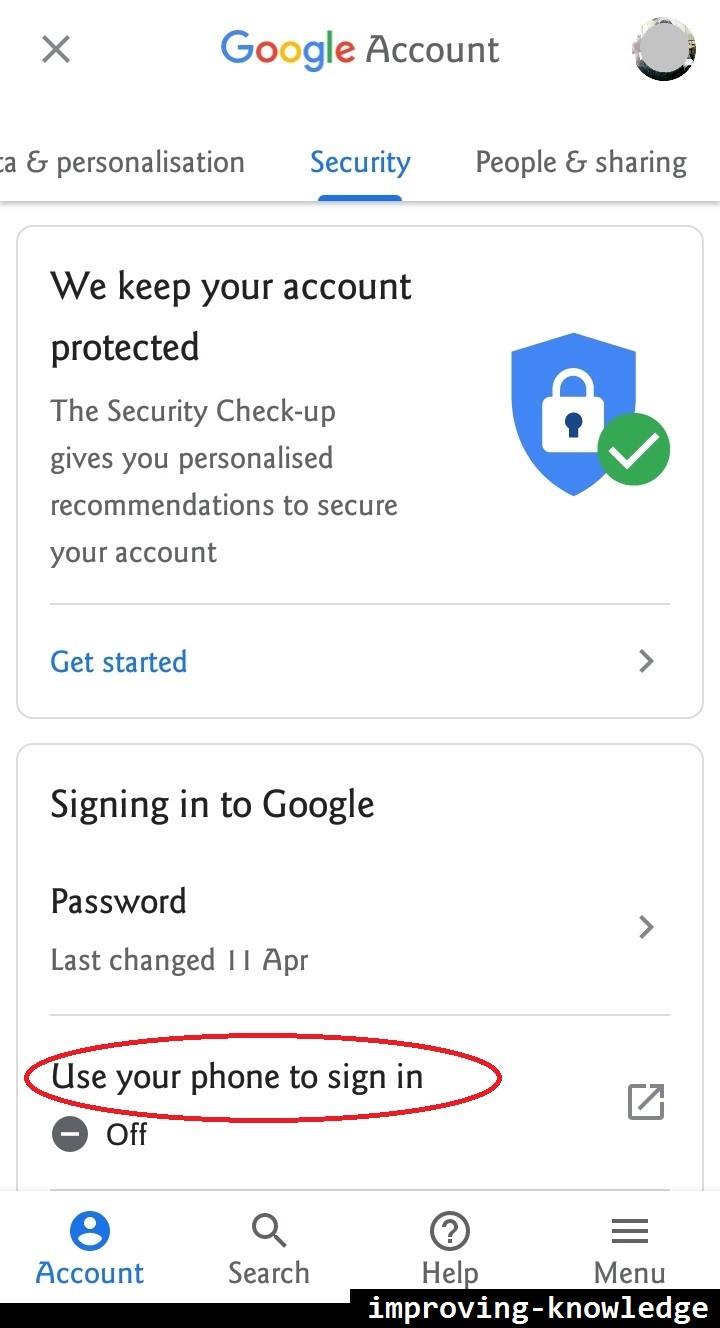This is a detailed screenshot of the Google Account security section. At the top left, there is an 'X' icon, followed by the Google logo, with each letter in its distinctive color: 'G' in blue, 'O' in red, 'O' in yellow, 'G' in blue, 'L' in green, and 'E' in red. Adjacent to the logo, it reads "Google Account" beside a blurred profile picture of the account holder.

Below this header, there are menu tabs labeled: "Home," "Personal info," "Data & personalization," "Security," "People & sharing," with "Security" highlighted in blue and underlined. The main section contains a statement, "We keep your account protected," followed by, "The Security Checkup gives you personalized recommendations to secure your account." To the right, there is an illustration comprising a blue shield with a lock and a green circle containing a white checkmark.

Beneath this section, a blue "Get Started" button with a 'greater than' symbol indicating a clickable link guides users to further options.

Further down, another box is visible, titled "Signing in to Google." Inside, it notes the password's last change date as "11 April," near another 'greater than' symbol. Below a dividing line, a section titled "Use your phone to sign in" shows a gray circle with a white minus sign labeled "Off." This section also contains a gray box with an upward-pointing arrow, and "Use your phone to sign in" is encircled in red.

Outside this main box, towards the bottom of the screenshot, a navigation bar includes "Account" (highlighted in blue), "Search" represented by a magnifying glass, "Help" indicated by a circled question mark, and an additional menu accessed by three horizontal lines. Finally, a black bar at the bottom reads "Improving knowledge."